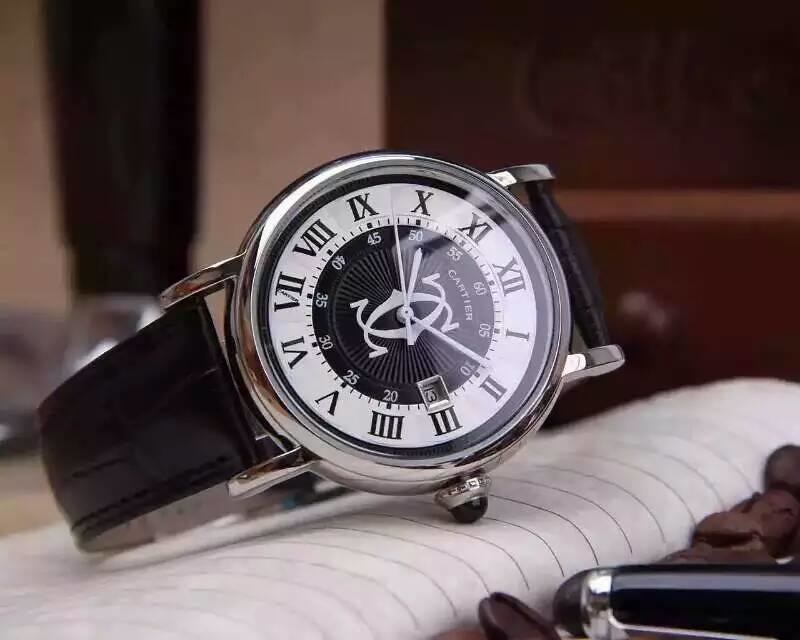This photograph showcases a luxurious Cartier wristwatch prominently displayed on a lined white notepad. The watch features a sleek black leather band, a white clock face with an inner black circle, and is adorned with silver-toned hardware. The timepiece's dial displays Roman numerals and elegantly crafted white hour, minute, and second hands, indicating a time of approximately 11:08 and 45 seconds. Visible in the center of the watch face is the distinguished Cartier branding accompanied by the iconic "C" logo. The background subtly includes elements of a wall, a dresser, and the tip of a ballpoint pen, adding context without detracting from the main subject.